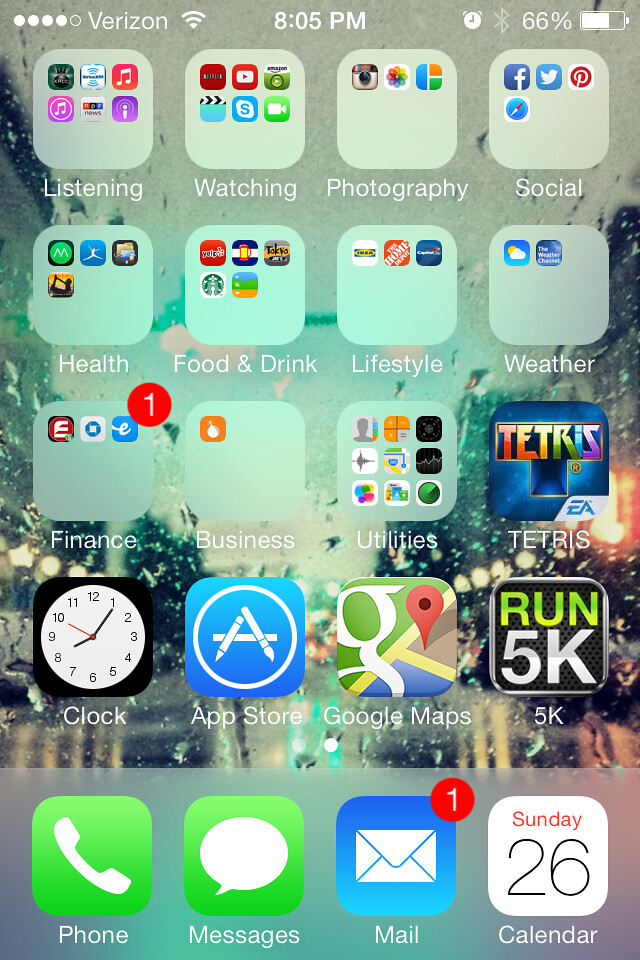**Detailed Description of the Image:**

The image is a vertically-oriented screenshot captured from a smartphone or tablet, with the screen showcasing various menus and software programs. The device is connected to the Verizon network, with the status indicators along the top displaying the time as 8:05 PM and the battery level at 66%. These indicators are in white text.

The interface features a series of light bluish-green square icons that categorize different types of information and functionalities available on the device. These categories include:

1. Listening
2. Watching
3. Photography
4. Social
5. Food and Drink
6. Lifestyle
7. Health
8. Weather
9. Finance
10. Business
11. Utilities

Additionally, the home screen includes specific applications such as Tetris, a clock showing the current time as 8:05 PM, the App Store, Google Maps, and a fitness app titled "Run 5K."

At the bottom row of the app icons, there are essential utilities including:
1. Telephone - represented by a green icon with a white silhouetted handset.
2. Messages - likely a text messaging app.
3. Mail - indicated by an envelope icon on a blue background, showing one unread message.

The date displayed on the calendar app is Sunday the 26th. The word "Sunday" is written in red with the number "26" in black.

All these icons and applications are shown against a background image depicting a cityscape, adding a dynamic visual element to the overall interface.

**End of Description**: This concludes the detailed description of the screen capture. Thank you for viewing and we hope you found this description helpful. See you in the next description!